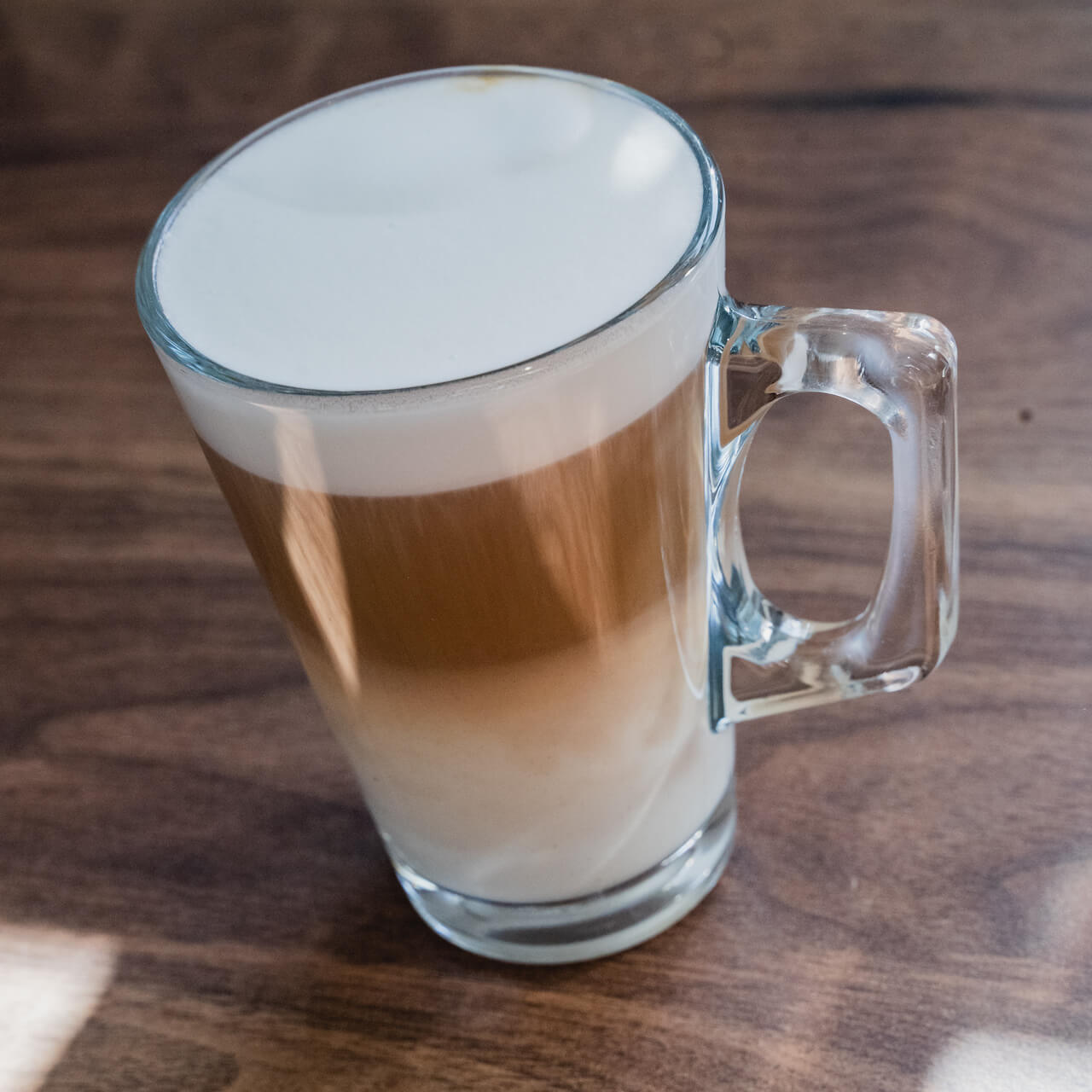This detailed point-of-view photograph captures a close-up of a clear glass mug filled with a multi-layered beverage, likely a coffee or latte-type drink, sitting on a wooden table. The image, taken from slightly above, highlights the distinct layers within the drink, under natural sunlight, hinting at a nearby window. The topmost layer consists of approximately half an inch of pure white foam, indicative of a frothy texture. Beneath the foam lies about two inches of a medium, rich, light brown liquid that suggests the presence of coffee. This middle layer gradually transitions into the bottom layer, which is a thicker, cream-colored liquid, implying an infusion of milk or cream. The clear, plain glass mug features a thick handle and offers an unobstructed view of the layered concoction within. The shared emphasis on the detailed structure and coloration of the beverage layers contributes to a comprehensive description of this inviting, likely coffee-based drink.